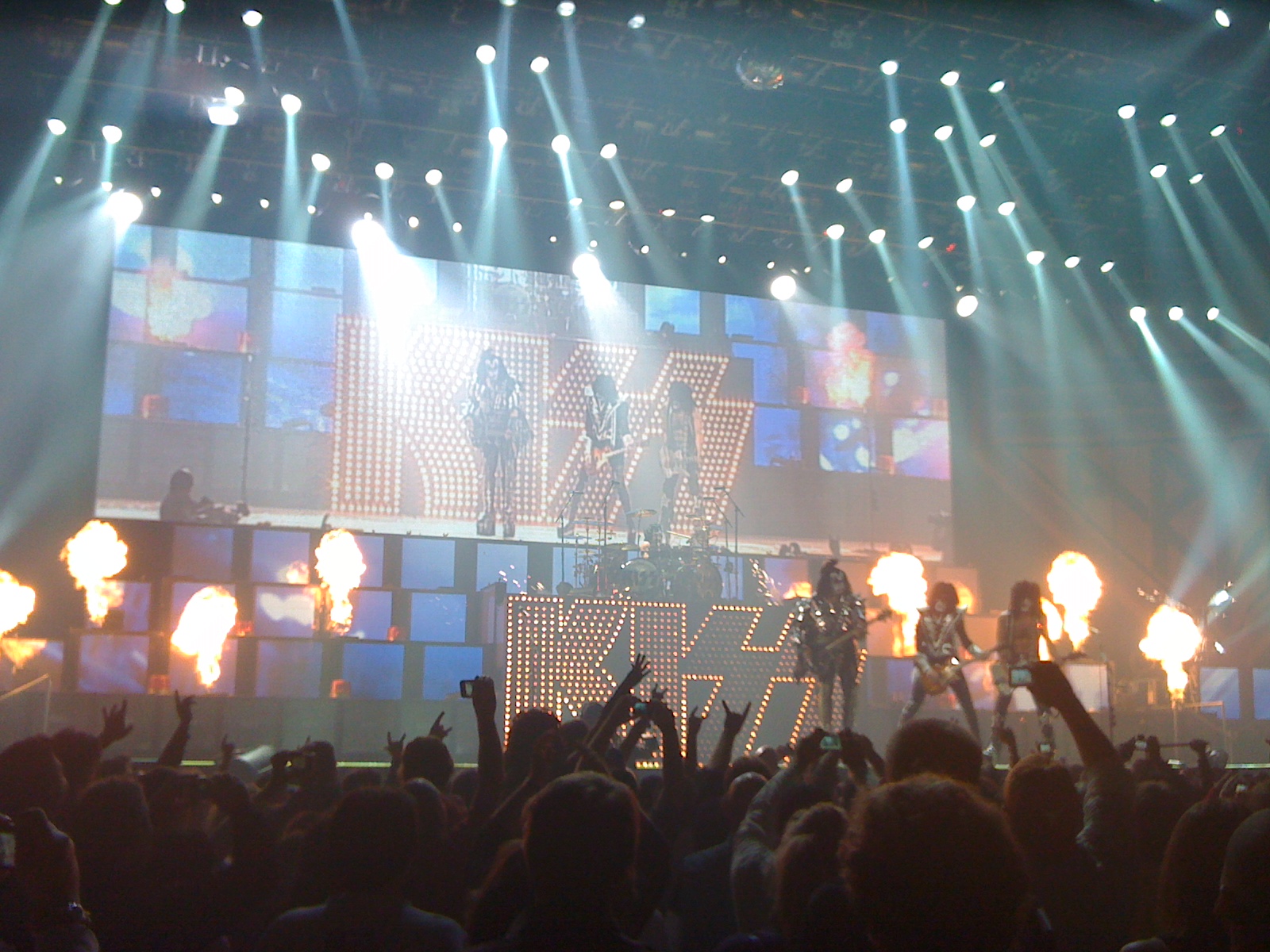This photograph captures the electrifying atmosphere of a KISS concert from the perspective of someone in the enthusiastic crowd. Up front, we see a sea of fans with their hands in the air, many holding up smartphones to capture the moment. The audience is dimly lit, making individual faces indistinguishable, but the excitement is palpable with numerous rock-and-roll hand signs and phone screens glowing.

Dominating the stage are the iconic band members: Gene Simmons, Ace Frehley, and Paul Stanley, clad in their signature black leather, towering platform boots, and unmistakable face paint. Each is wielding a guitar or bass, completely immersed in their performance. Behind them, sitting elevated on a drum set atop a platform emblazoned with the illuminated KISS logo, is the drummer, likely Peter Criss, partially obscured but energetically keeping the beat.

Adding to the spectacle, a large jumbotron screen projects bigger-than-life images of the performers, ensuring that even those at the far ends of the extensive crowd can see the details of the show. The stage is bathed in intense lighting from a myriad of spotlights, casting a blue haze over the scene, while bright orange flames shoot up at various points, creating a thrilling pyrotechnic display that frames the band spectacularly.

The KISS logo, outlined with tight gold lights and bursting with visual energy, anchors the stage scenery, while the dramatic lighting and pyrotechnics contribute to the grandiosity. The combination of the band's dynamic presence, the roaring flames, and the lights makes for a vivid, unforgettable concert photograph that encapsulates the raw energy and larger-than-life persona of a KISS performance.